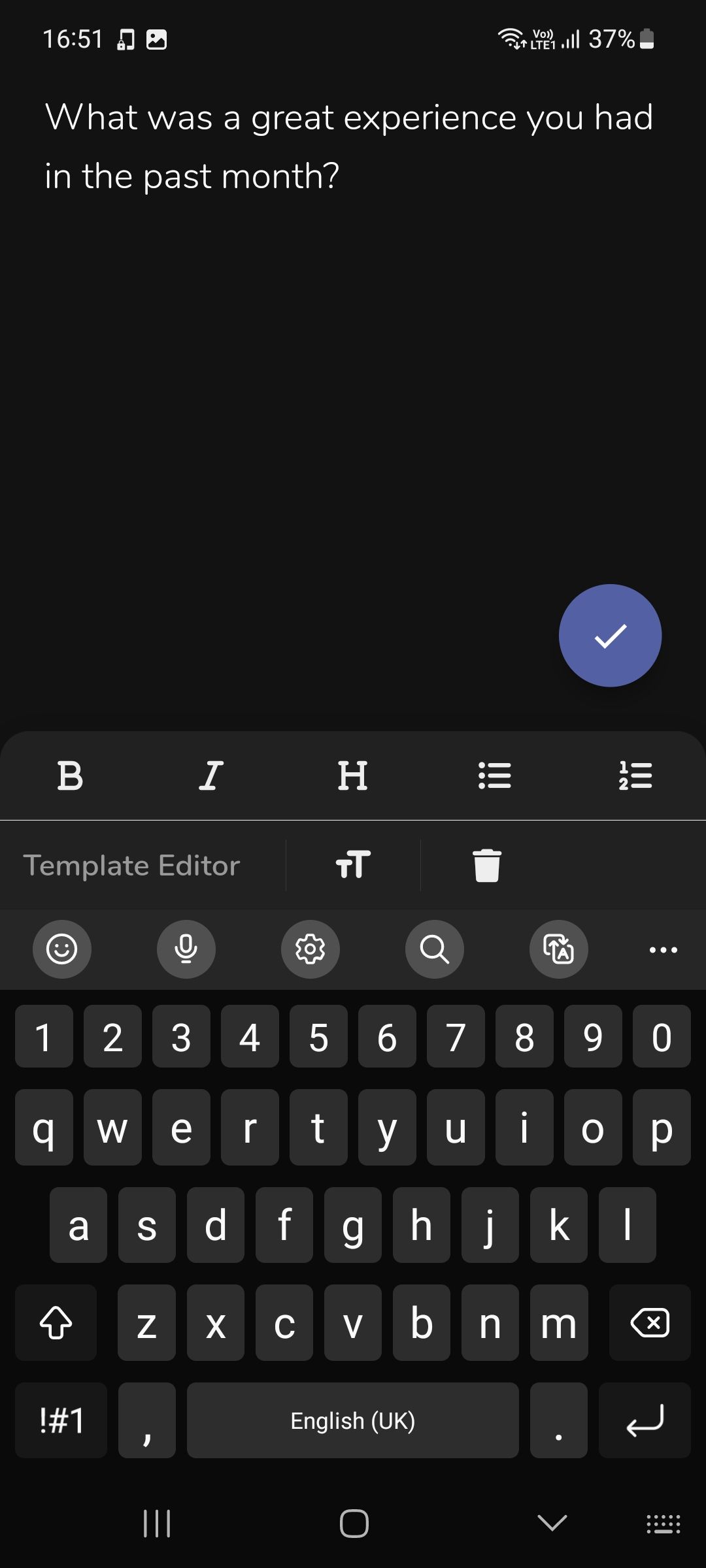Here is a cleaned-up, detailed caption for the smartphone screenshot:

---

The screenshot displays a smartphone interface with a black background and white text at the top. The top bar shows a timestamp reading "16:51" alongside several icons: a lock screen icon, a picture/icon grid, a Wi-Fi signal indicator, an LTE connection symbol, and a battery icon showing 37% charge. Below this, text prompts the user with the question, "What was the great experience you had in the past month?"

Further down, there is ample black space leading to a prominent purple circle with a white check mark inside. Below this circle, there are several formatting option tabs, including bold, font adjustments, uppercase/lowercase toggles, bullet points, and numbering. Beneath these tabs is a faint gray line labeled "Template Editor."

Continuing down, another set of icons is displayed: a small "T" with a low checkmark (unidentified function), followed by a trash can icon. 

At the very bottom, a horizontal bar includes a smiley face emoji, a microphone icon, a settings gear, a search icon, an unknown icon featuring two arrow-formed boxes next to three horizontal dots, and a full-screen keyboard layout. The screen's keyboard itself occupies the lowest portion of the screenshot. Below this keyboard are navigation and function buttons: a close down button, a home button, a drop-down arrow, and a screen keyboard icon.

---

This description provides an organized and detailed overview of the various elements visible in the smartphone screenshot.